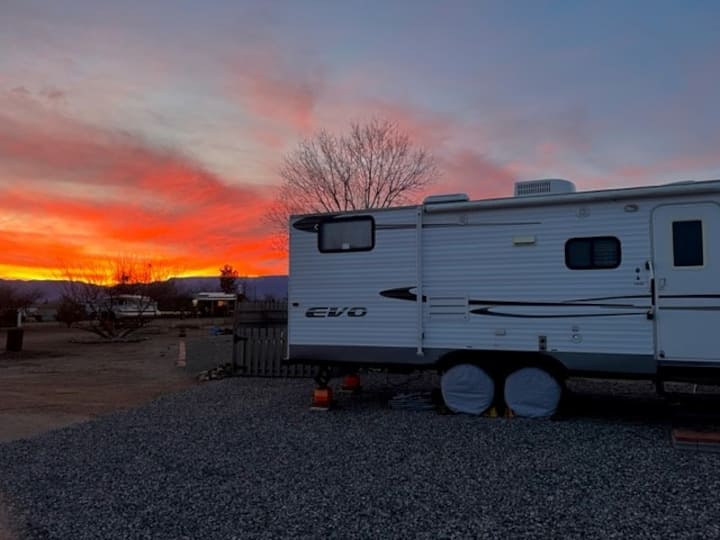The image depicts a large, white camper with the brand name "Evo" prominently displayed in black text on the back. Two black lines run across its rear. The camper, which appears expensive, is stationed on a gravelly surface with orange blocks supporting its wheels, indicating it is not hooked up to a vehicle. The wheels have protective covers or cloths, emphasizing that it is not currently in use. A wooden fence sits beside it and a tree without leaves stands behind, with additional leafless trees visible to the left, suggesting a fall or winter setting. Beyond the camper, there are hints of other vehicles, but no buildings are visible. The background features majestic mountains and a stunning sunset, blending hues of orange, yellow, and dim blue under a slightly cloudy sky, adding a serene and picturesque element to the scene.